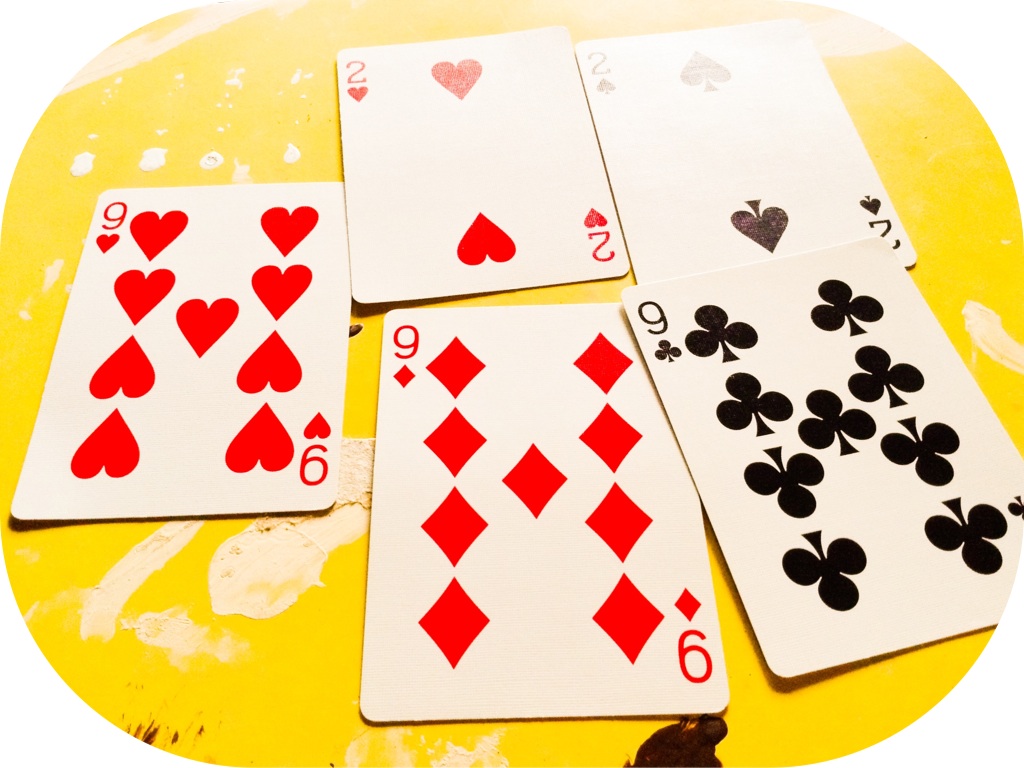A captivating image showcases a close-up of four playing cards, suggesting a game of poker in progress. The cards, meticulously arranged on a vibrant yellow table with artistic white and black paint splatters, prominently feature a full house combination: the nine of hearts (red), the nine of diamonds (red), the nine of clubs (black), the two of hearts (red), and the two of spades (black). The image is creatively framed with deep rounded corners and contains no text. The foreground is dominated by the cards, which occupy approximately 95% of the photo's space, emphasizing their importance in the composition. No individuals are present, allowing the viewer to fully appreciate the intricate details and vivid colors of the cards and their backdrop.